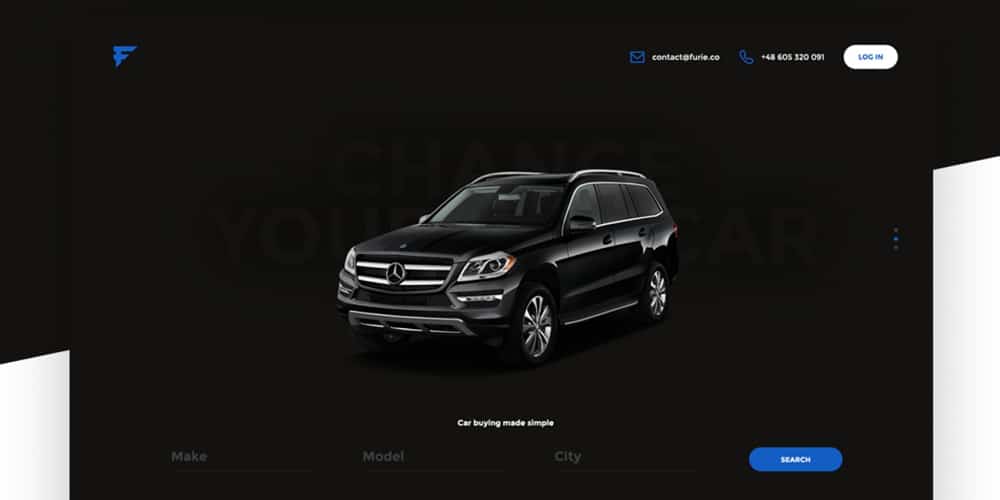A screenshot features a sleek black Mercedes-Benz SUV, prominently displayed in the center, facing slightly toward the left. The vehicle shines against a completely black background, emphasizing its elegant design and silver rims. In the upper left corner, a blue "F" logo is visible, possibly indicating the brand or website. On the far right side of the screen, there are several icons: a link to a website, a telephone icon followed by a phone number, and a login button. At the bottom, a horizontal menu includes options labeled "MEEC," "Model," "City," and a blue "Search" button with white text. Above these options, white text reads "Carbine Made Simple," underscoring the focus of the page. The overall layout is clean and user-friendly, emphasizing the luxury SUV and easy navigation options.